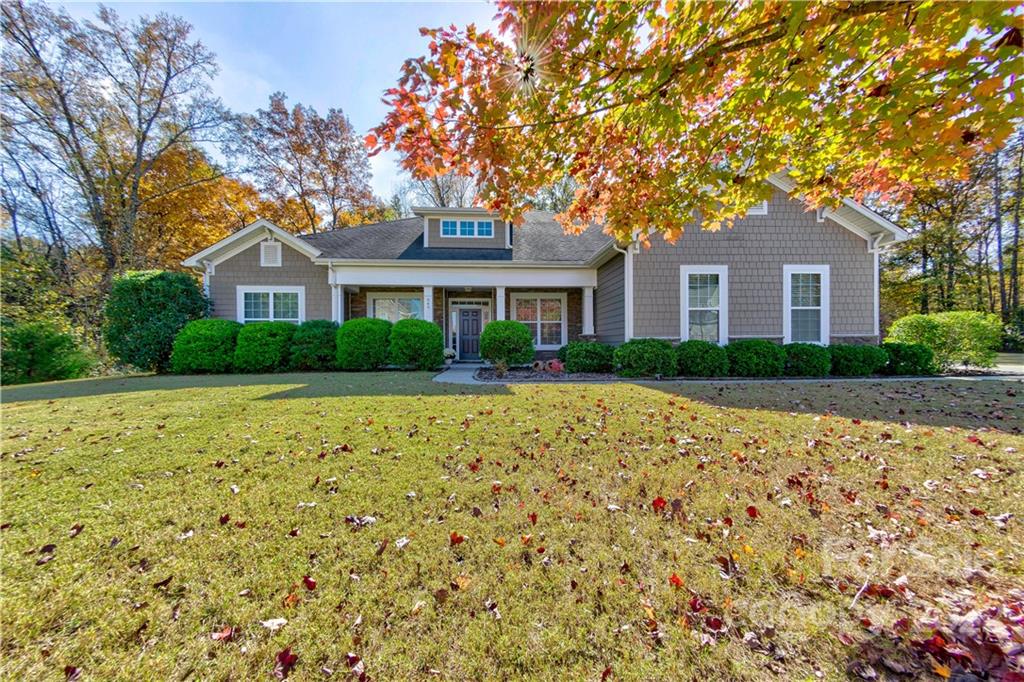In this detailed daytime photograph, we see a charming suburban, single-story house with a small loft area situated in a picturesque neighborhood. The house, painted a dark gray with white wooden siding, features a welcoming front porch with four white pillars and a dark wooden door flanked by white-framed windows. The roof, possibly made of black asphalt shingles, includes white soffit vents and a couple of louver vents.

Surrounding the house is a meticulously maintained front yard with a green, freshly cut lawn scattered with fallen leaves in shades of red, brown, and yellow, indicating the autumn season. The landscaping includes numerous green shrubs, with five clustered together and one particularly tall shrub standing out. A curved sidewalk, transitioning from the driveway to the front door, adds a graceful touch to the scene.

Tall, mature trees with a mix of bare branches and some retaining their fall-colored leaves provide a serene backdrop. To the right of the house, more trees and shrubs extend along the sidewalk, enhancing the suburban ambiance. The bright blue sky with occasional clouds completes this picturesque autumn setting.